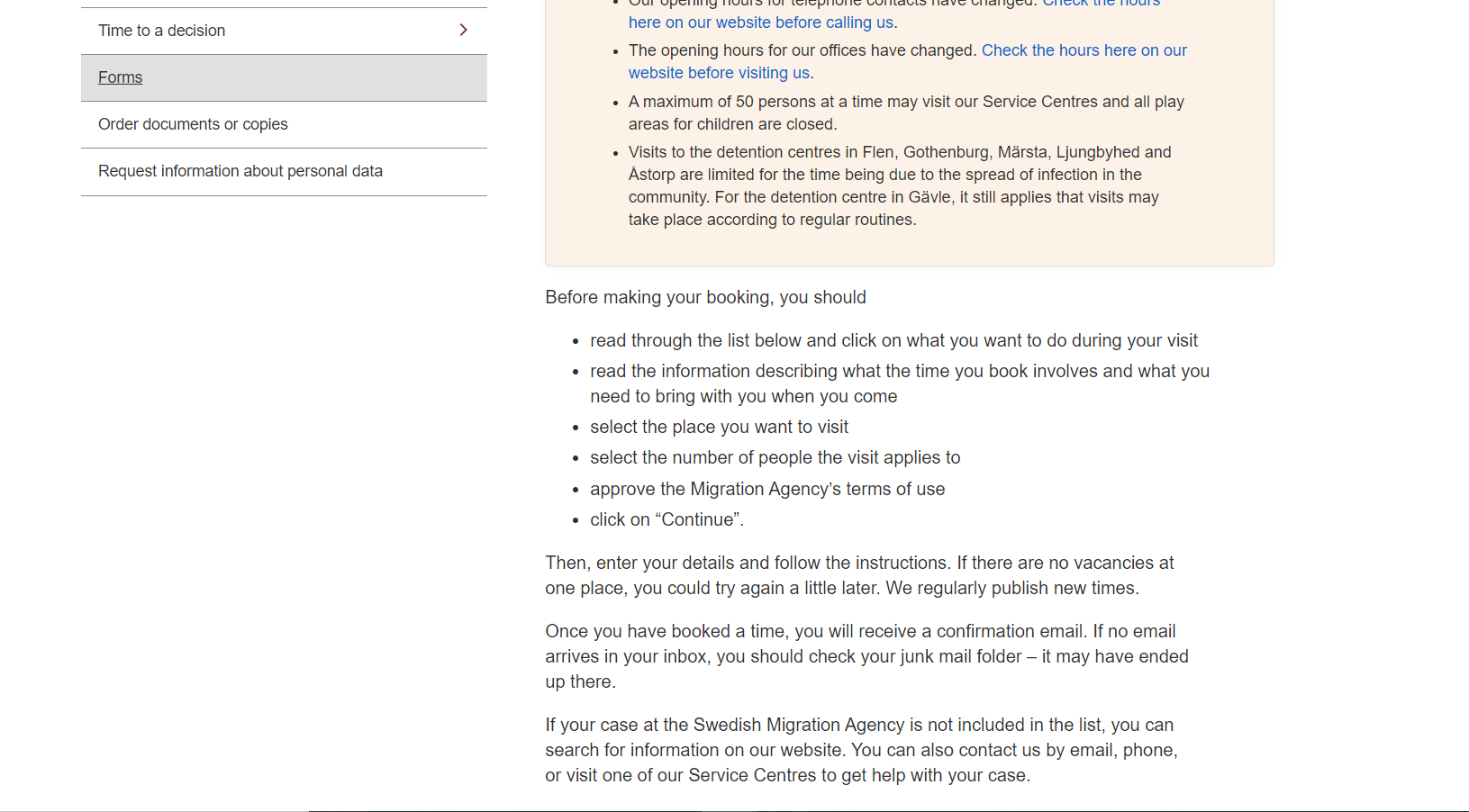The image appears to be a detailed screenshot of an official website providing information about various services and updates. 

On the left side of the webpage, there is a navigation pane consisting of several sections: 
1. "Time to a Decision" with an arrow pointing to the right.
2. A clickable, underlined link labeled "Forms," which includes options to order documents or copies, and request information about personal data.

On the right side, there are several sections of important announcements and instructions:

1. **Notice about Office Hours**:
   - "The opening hours for our offices have changed. Check the hours here on our website before visiting us."
   - "A maximum of 50 persons at a time may visit our service centers, and all play areas for children are closed."
   - "Visits to the detention centers in Phlegm, Gothenburg, Marsta, Jungwiad, and Astorp are limited for the time being due to the spread of infection in the community."
   - "For the detention center in Gabi, it still applies that visits may take place according to regular routines."

2. **Booking Instructions**:
   - A section begins with the heading, "Before your booking, you should," followed by six bullet points presumably providing detailed pre-booking guidelines.
   - Below that, instructions state, "Then enter your details and follow the instructions. If there are no vacancies at one place, you could try again a little later. We regularly publish new times."

The webpage seems to be from an organization managing appointments or visits, possibly in a government or community services context, offering detailed instructions and updates regarding their operations during health safety measures.